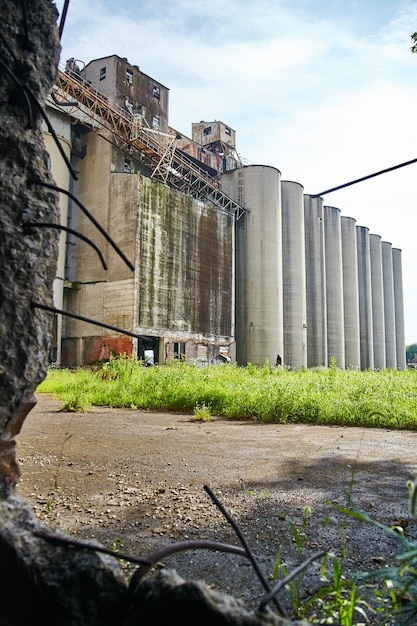This is a detailed photograph of an abandoned industrial facility, likely an old factory or manufacturing plant, set against a backdrop of a blue sky filled with clouds. The central focus is a large, weathered building with a rectangular shape, characterized by its aged and rusted cement walls, broken windows, and scaffolding indicating possible ongoing or unfinished renovation. On the front-left side of the building, steel rebar juts out from broken, moss-covered concrete, while on the right side, nine cylindrical silos rise about five stories tall, appearing white or gray, likely used previously for storing liquids or other materials.

In the foreground of the image, scattered debris and broken concrete pieces can be seen, through which an expanse of gravel or paved driveway leads to the overgrown grass. A watchtower, a cube-like structure with windows, can be observed on top of the building, suggesting it once served a supervisory role. One open door on the ground floor allows a view through the structure, highlighting its hollow and unused state, and giving a sense of desolation. A collapsed steel bridge or scaffold leans against the building, adding to the impression of neglect. Unkempt grass has grown around the facility, emphasized by the dirt-covered ground and concrete remnants scattered about. The overall scene suggests a once-bustling industrial hub now left to decay, far removed from the busyness of urban life.